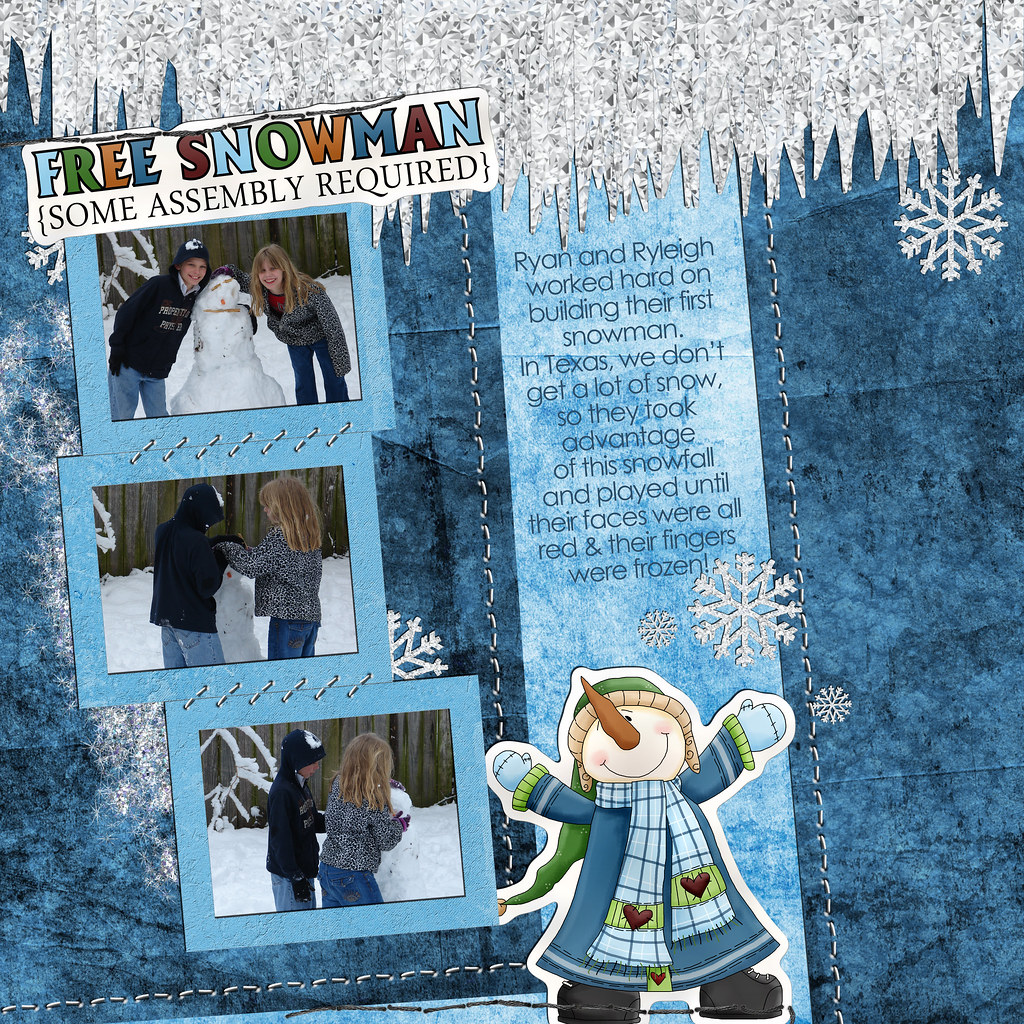In this image, a playful, winter-themed design is set against a rich blue backdrop with scattered white snowflakes and textured white icicles hanging down from the top. On the left side, three photos depict a young girl and boy, Ryan and Riley, busily building a snowman. The bottom-left photo shows them starting the process, the middle photo captures them working in full swing, while the top photo reveals their completed snowman masterpiece. Above these photos, bold, multi-colored text reads "FREE SNOWMAN," followed by smaller, black text stating, "Some assembly required." To the bottom right, an animated snowman, donning a jacket and a heart-patterned scarf with a carrot nose, adds a whimsical touch. Blue text near this character reads, "Ryan and Riley worked hard on building their first snowman in Texas. We don't get a lot of snow, so they took advantage of this snowfall and played until their faces were red and their fingers were frozen."